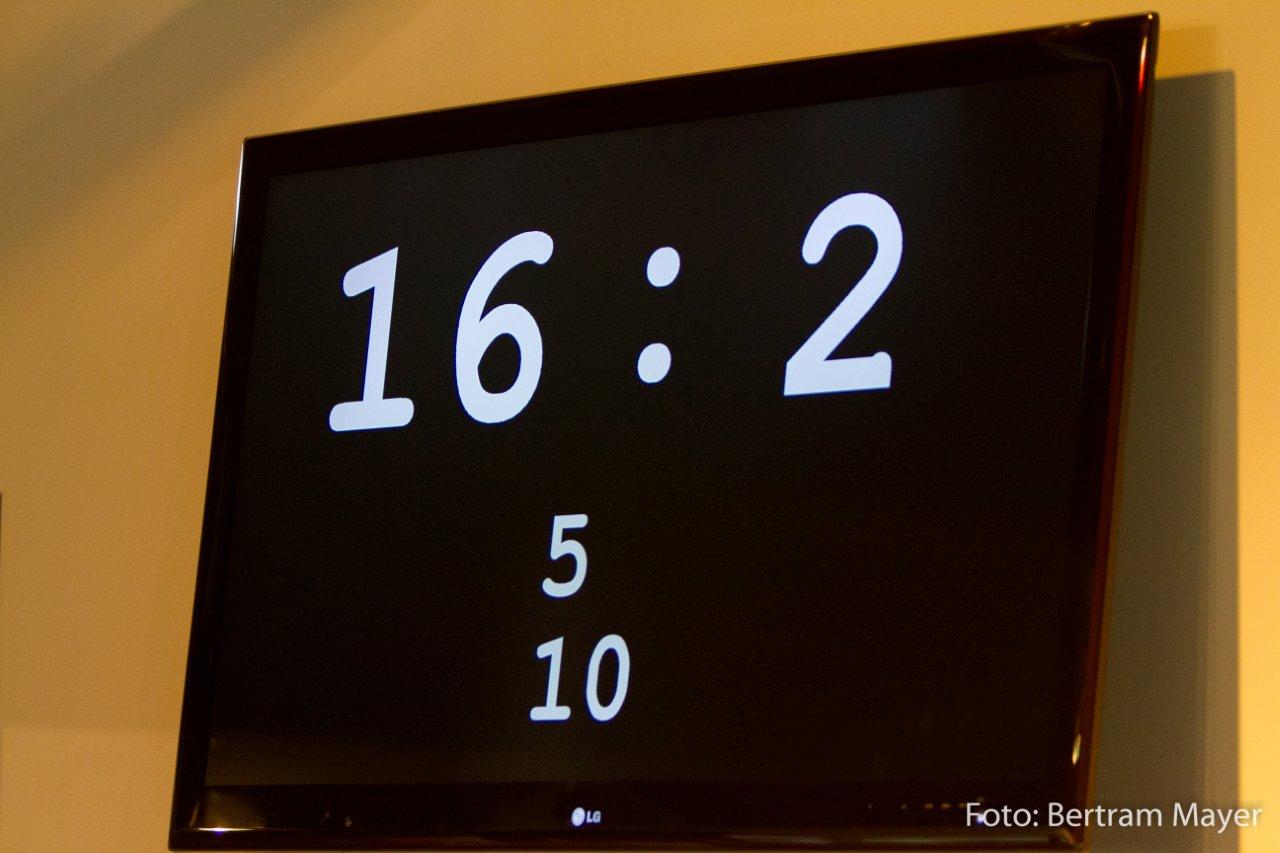In the image, there is a large, wall-mounted LG television with a black bezel reflected on a mustard-yellow wall. The screen displays white numbers: "16:2" at the top, followed by "5" directly underneath, and "10" below that. In the bottom corner of the image, there is a caption that reads "PHOTO: BERTRAM MAYER." The television appears quite wide and has noticeable shadows cast on the wall behind it, suggesting it is an older model with thicker bezels. The photo seems to have been taken with a mobile phone, not by a professional photographer.